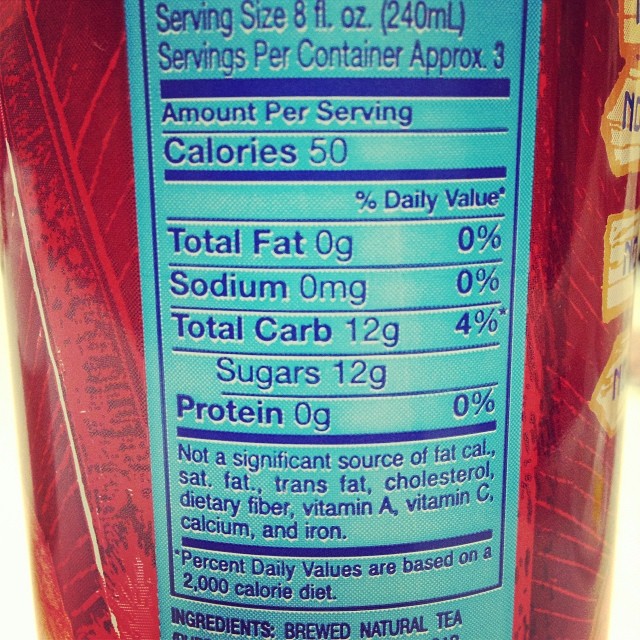This image is a close-up of the nutritional label on a red can, likely holding some kind of tea. The can itself is a deep, almost maroon red, decorated with a subtle pattern of tan lines that resemble wood graphics, barely visible on the right edge. The label for the nutritional information is a turquoise or cyan blue with dark blue text. It states the serving size as 8 fluid ounces (240 ml) with approximately 3 servings per container, totaling 24 fluid ounces of liquid. The label details per serving: 50 calories, 0 grams of fat (0%), 0 milligrams of sodium (0%), 12 grams of carbohydrates (4%), 12 grams of sugar, and 0 grams of protein (0%). It also notes that it is not a significant source of fat, calories, saturated fat, trans fat, cholesterol, dietary fiber, vitamin A, vitamin C, calcium, and iron, and that the percent daily values are based on a 2000 calorie diet. At the bottom of the label, though partially cut off, it indicates the ingredients include brewed natural tea.